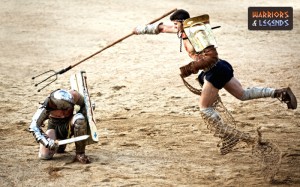In this professionally shot, full-color outdoor photograph, natural light illuminates a dramatic gladiatorial combat scene set against a simple backdrop of brown sand, pockmarked with numerous footprints. The image, rectangular in shape and without border, features a black rectangle in the upper right corner bearing the title "Warriors" in red and "Andalegians" in blue.

At the heart of the scene are two men engaged in fierce battle. On the right, a man who appears to be leaping or lunging forward, clad in minimal but striking combat gear: black shorts, tall white socks, and golden shoulder armor. He wields a long, menacing trident in one hand, raised high over his opponent, and a net is visible near his feet. In contrast, his opponent, crouching defensively on the left, wears comprehensive silver armor, including a helmet, gauntlets, and leg guards. He grips a shield firmly in one hand and a sword in the other, using the shield to protect himself from the imminent strike of the trident just above his head. The stark composition of sand and combatants captures a vivid moment of tension and action.